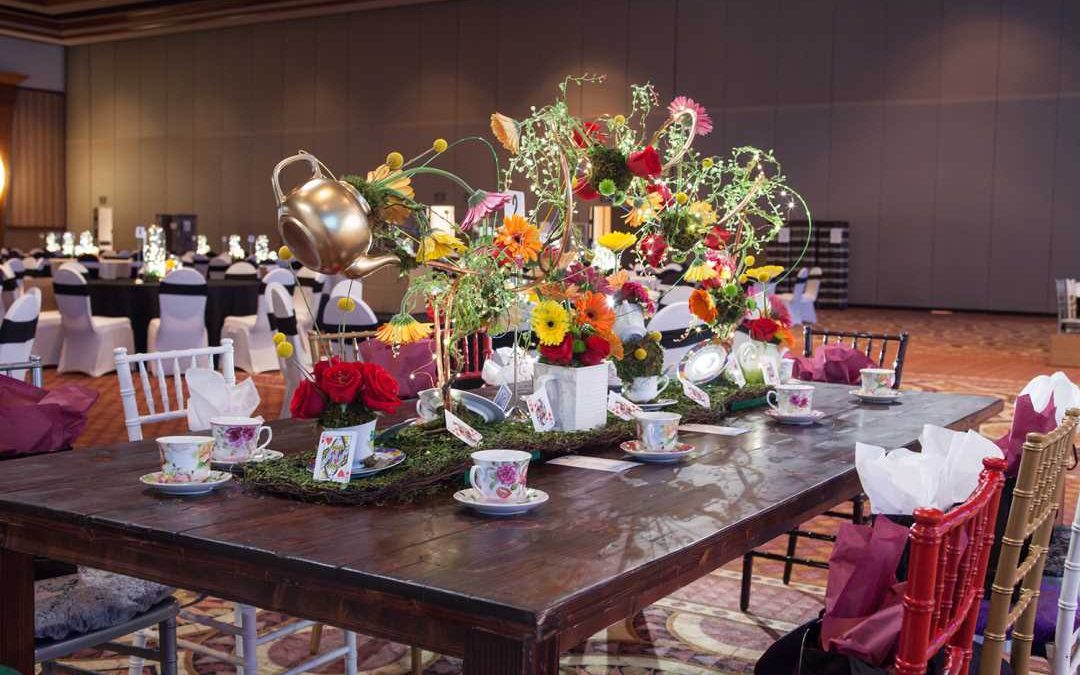This image showcases a vibrant Alice in Wonderland-themed banquet setup within a spacious hall with tall ceilings. A large, dark-stained wooden table is prominently featured in the foreground, surrounded by an eclectic mix of wooden chairs in red, brown, white, and black hues. Each chair holds a purple goody bag, adding an element of surprise and whimsy.

Dominating the center of the table is an elaborate centerpiece: a long rectangular tray filled with colorful flowers and lush green grass, nearly covering the table's surface. Complementing this floral display are playful decorations, including teacups with dainty floral patterns positioned at each seat, and a golden teapot designed to appear as though it is charmingly spilling flowers and plants across the table. Interspersed among the plants are whimsical playing cards, further enhancing the Alice in Wonderland theme.

This particular table stands out from the rest in the venue, as the background reveals standard tables and chairs typical of a hotel conference room setting. The attention to detail in the decorations, from the teacups to the playing cards, creates an enchanting and immersive experience, distinctively setting the scene for a magical event.